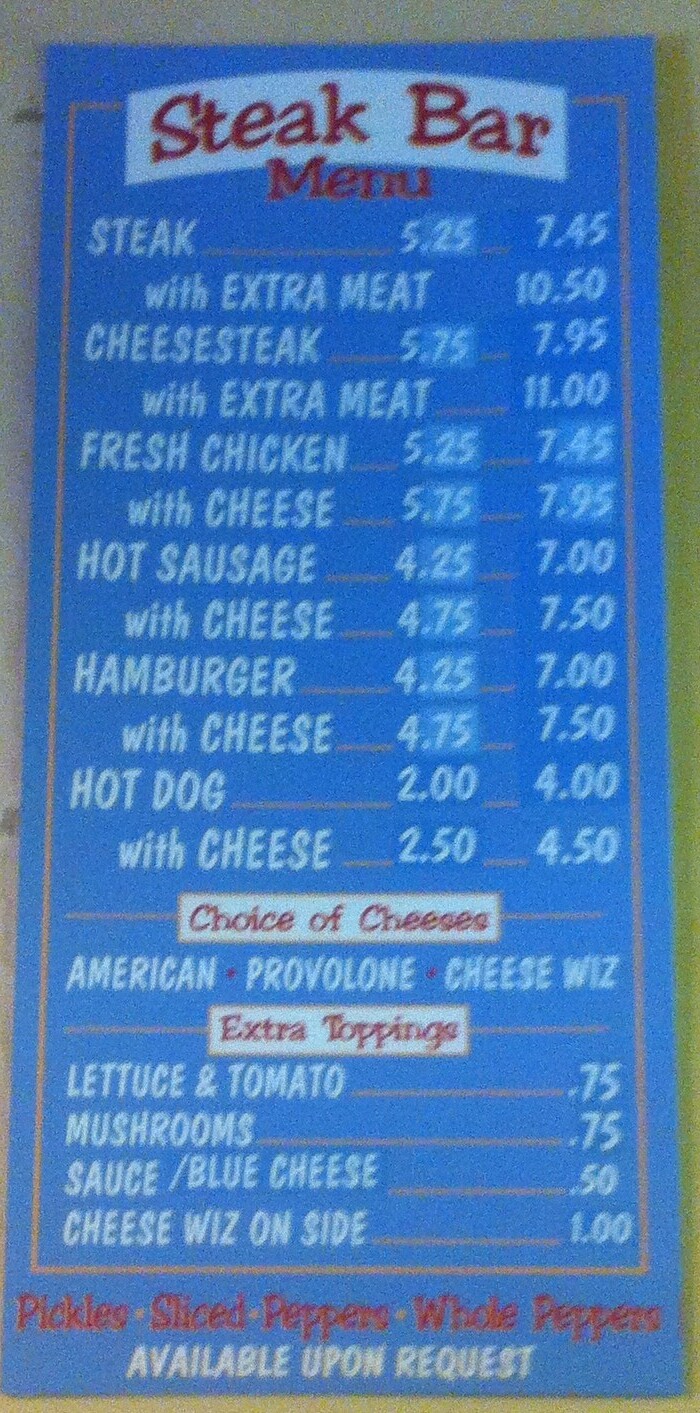This image showcases a rectangular menu board with a blue backdrop and a neutral, brownish border framing the food choices. The top of the menu features a white banner with "Steak Bar Menu" prominently displayed in red lettering. Below this, an array of delectable options is listed, including Steak with Extra Meat, Cheesesteak with Extra Meat, Fresh Chicken with Cheese, Hot Sausage, Hamburger, and Hot Dog, all of which come with cheese options.

The menu details the available cheese choices—American, Provolone, and Cheez Whiz—in a white rectangular box with red lettering. Another white box with red lettering lists various extra toppings. At the very bottom, the menu notes that pickles, sliced peppers, and whole peppers are available upon request, marked in red lettering with a white font. The entire menu is mounted on a wall, and prices are clearly displayed next to each item.